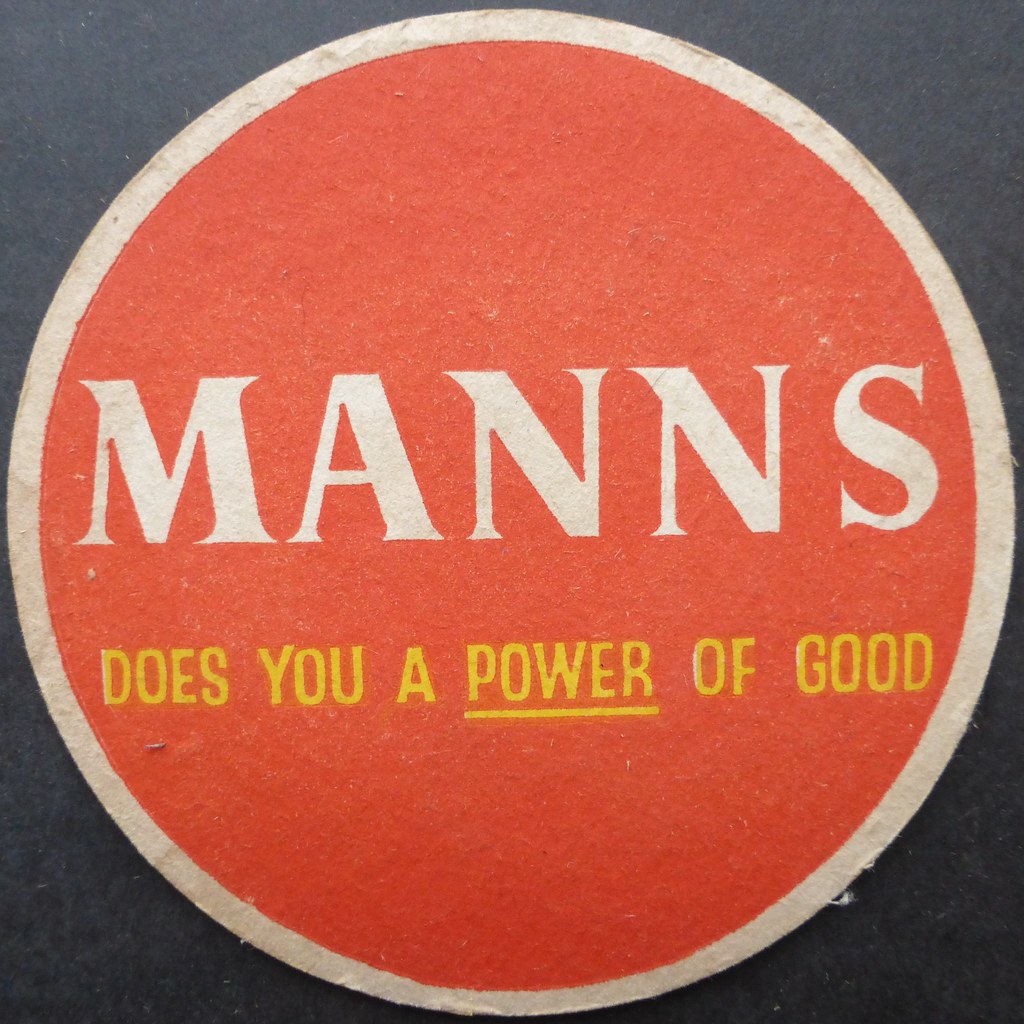The image depicts an old advertisement sign, characterized by its gritty, textured design reminiscent of aged paper. The background is a nearly black, charcoal gray square, visible mostly in the corners. Dominating the center is a large red circle with a white border. The circle features the bold white letters "MANS" in all caps, and below, in smaller yellow all-cap letters, the slogan "DOES YOU A POWER OF GOOD," with the word "POWER" underlined in yellow. The overall shading gives the impression of a slightly brighter top fading into a darker bottom, enhancing the vintage feel of the advertisement.